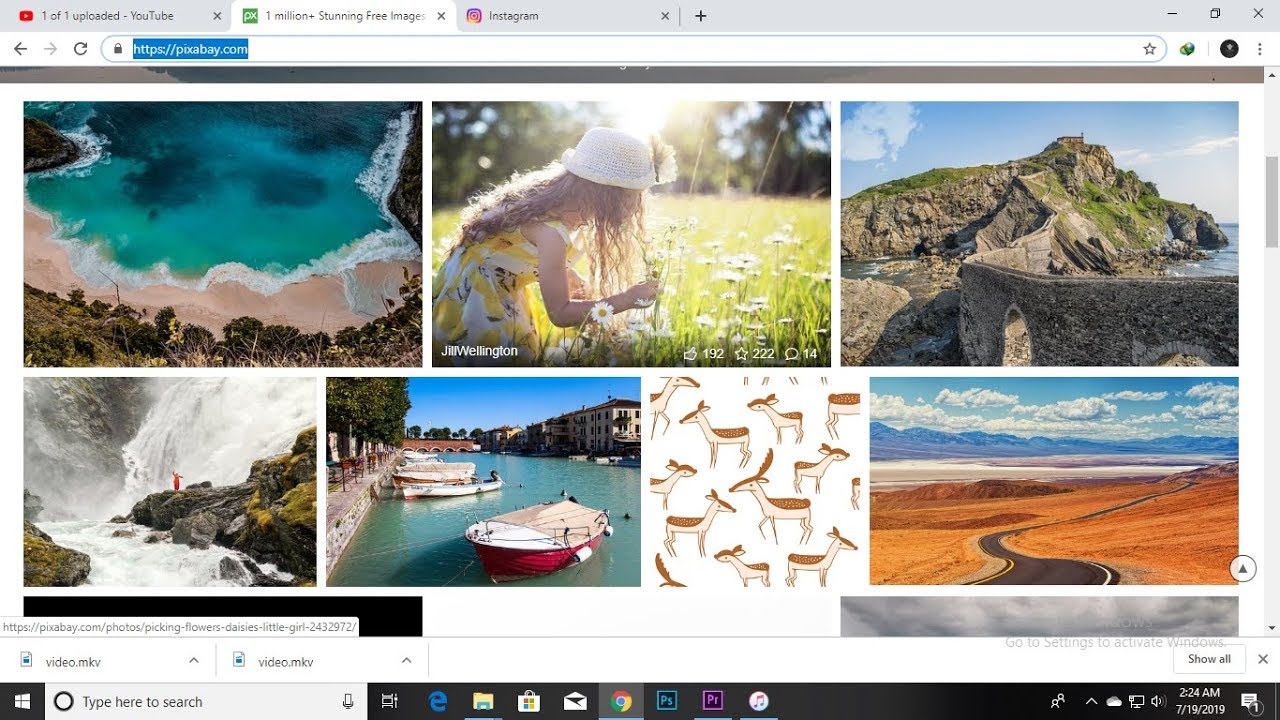The image depicts a web page from the website "https://pixabay.com," highlighted in blue in the upper left corner. The web page is designed as a collage, showcasing a series of images arranged in two distinct rows. The top row features three images: the first image captures an idyllic seashore with crystalline blue water and a sandy coastline; the second image portrays a side profile of a young girl in a yellow dress, long brown hair, and a white hat, picking sunflowers in a verdant grassy field under the sunny sky; the third image reveals a rugged seashore with prominent rocky formations and a stone wall. The bottom row houses four additional images, making the collage an engaging visual spread.